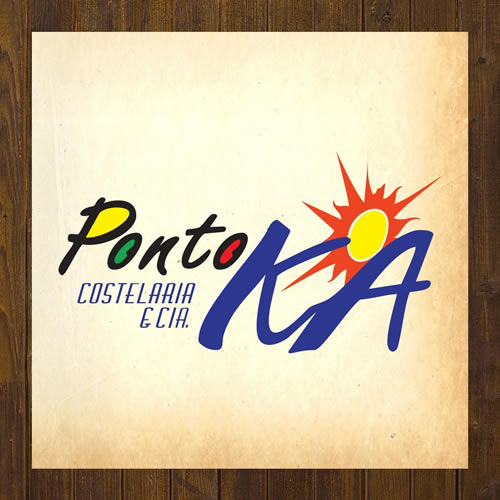The image features a colorful, detailed advertisement set against a wood grain background, perhaps resembling a table in a bar setting. In the center of the composition is a piece of tan parchment-like paper. Prominently displayed is the word "PONTO," with the letters filled with vibrant colors: the P is yellow, the first O is green, and the second O is red. Below "PONTO" is the phrase "KOSCHALAYA ISIA" written in blue cursive text. Positioned to the right is the abbreviation "K-A" also in blue, with a sun emblem behind it. The sun has a yellow center and orange rays extending outward, blending into a reddish-brown border surrounding the image. The overall background shifts between white and reddish-brown hues, giving the ad a dynamic and inviting appearance.